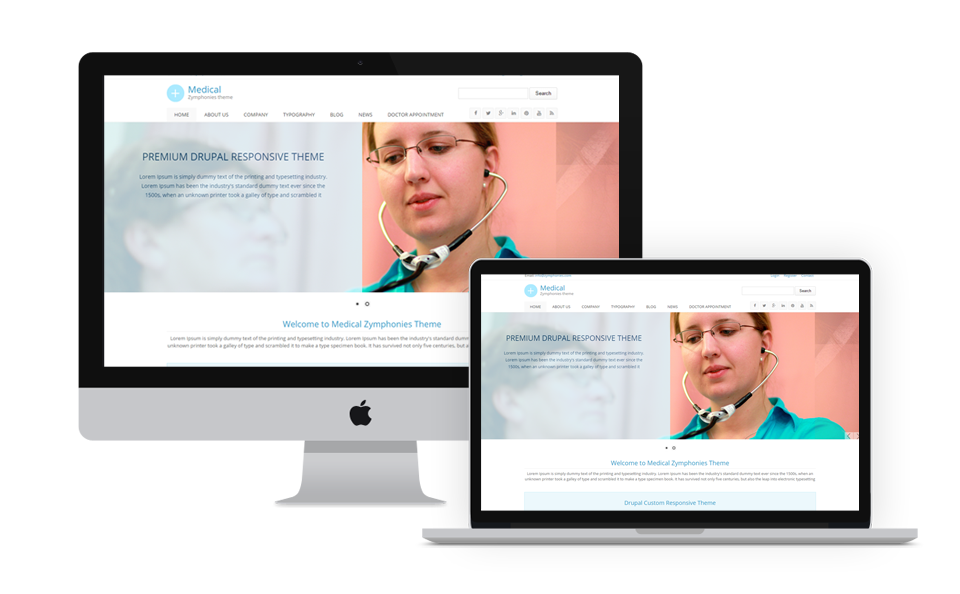In this image, we see both a desktop Mac and a MacBook, each displaying identical content on their screens. The screen shows a webpage featuring several navigation links, including Home, About Us, Company, Typography, Blog, News, and Doctor Appointment. Additionally, social media icons for Facebook, Twitter, Google Plus, and LinkedIn are visible. There is also a search bar prominently displayed. 

The webpage appears to be promoting a "Premium Drupal Response Theme." A portion of placeholder text, "Learn Ipsum is simply dummy text of the printing and typesetting industry, Learn Ipsum has been the industry's," is displayed, mimicking real content formatting. The scene suggests a modern, cohesive design layout suitable for various digital devices.